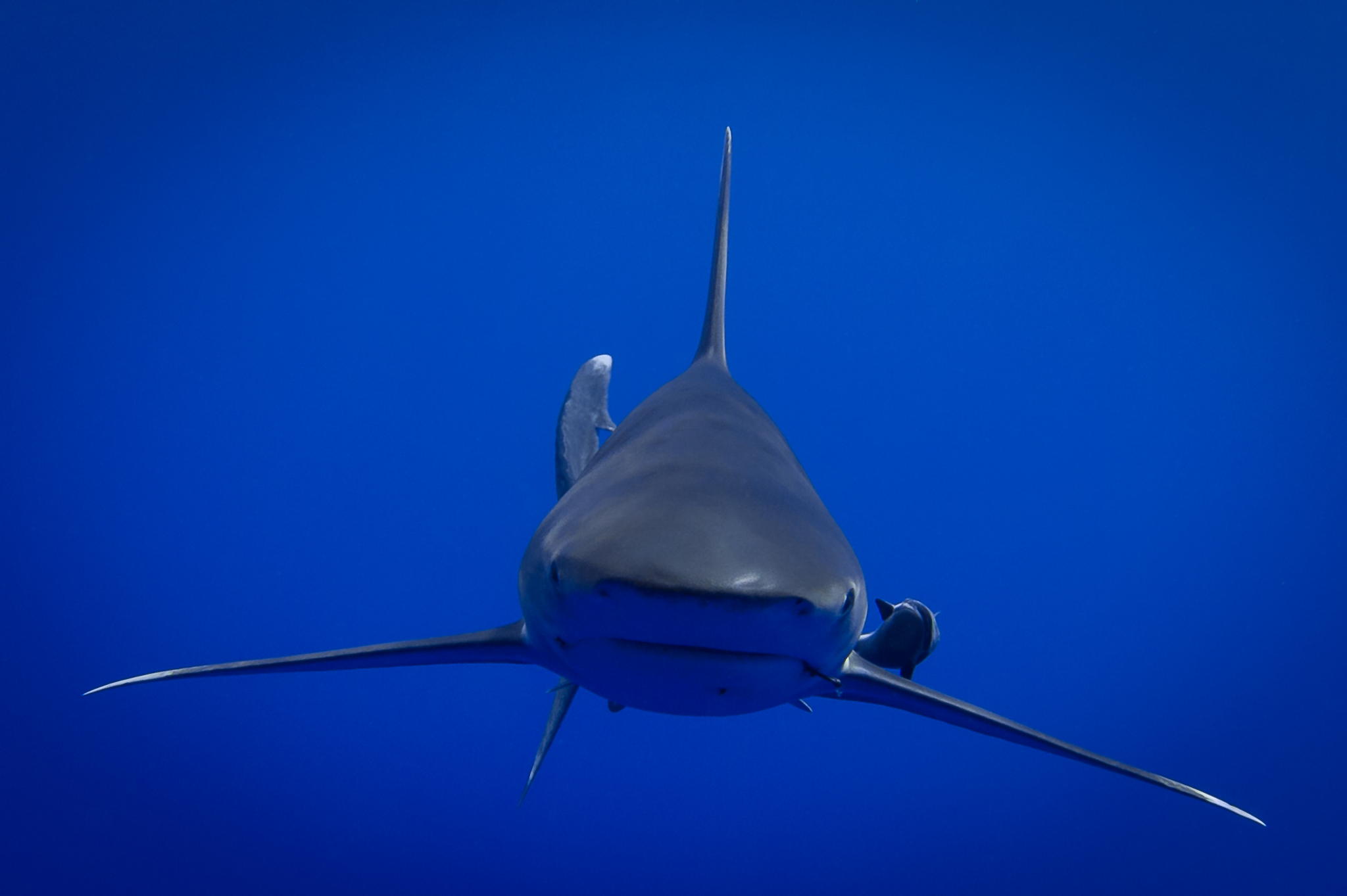This is a close-up photograph of a large bull shark swimming directly towards the camera, creating an intense and captivating front-on view. The shark's body resembles an airplane with its very pointy, gray nose and triangular shape. It has short but wide pectoral fins extending to either side, almost parallel to each other, and a tall, straight dorsal fin rising prominently from its back. The top of the shark is a typical dark gray, while the underside, including the area around its mouth, is a stark white. The dark, deep blue water surrounds the bull shark, enhancing its imposing presence. Off to the shark’s side, there appears to be a smaller fish or potentially a baby bull shark swimming nearby. The shark's eyes are fixed straight ahead, adding to the dramatic impact of the image.